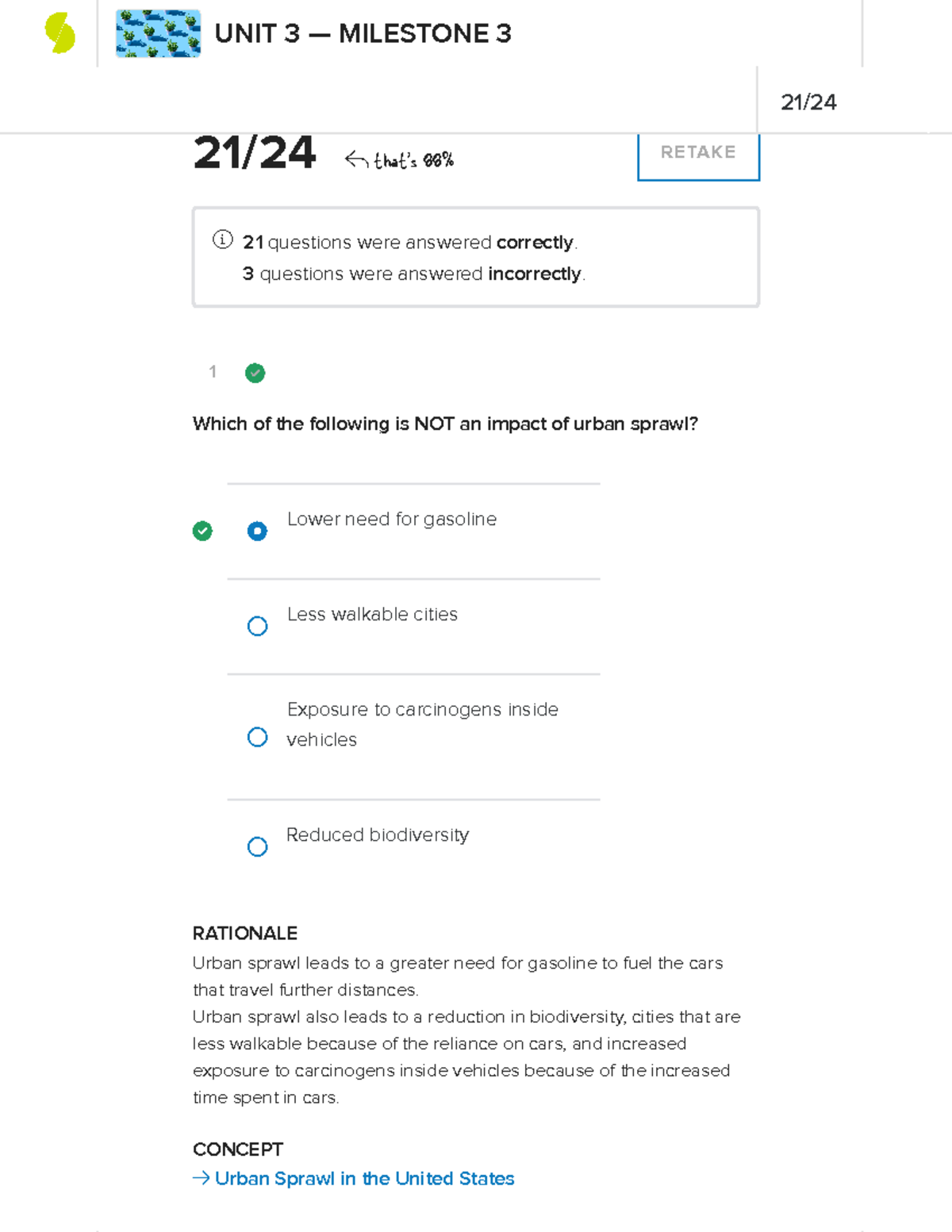The image displays the results of a test titled "Unit 3 Milestone 3." At the top left, the date "21/24" is noted, along with a score of "21/24," which equates to "88%," indicated to the right of the score. A button labeled "Retakes" is positioned on the right side. Below the score information, it clarifies that "21 questions were answered correctly" while "3 questions were answered incorrectly."

The question highlighted in the image asks, "Which of the following is **not** an impact of urban sprawl?" Four answers are provided:
1. Lower need for gasoline
2. Less walkable cities
3. Increased exposure to carcinogens inside vehicles
4. Reduced biodiversity

The user selected "Lower need for gasoline" as their answer. The explanation below indicates that urban sprawl actually leads to a greater need for gasoline to fuel cars traveling longer distances. Additionally, urban sprawl causes cities to become less walkable, reduces biodiversity, and increases exposure to carcinogens inside vehicles due to the extended time spent in cars.

The concept, "Urban Sprawl in the United States," is highlighted at the bottom, with its text color in blue, contrasting against the predominantly black text on a white background.